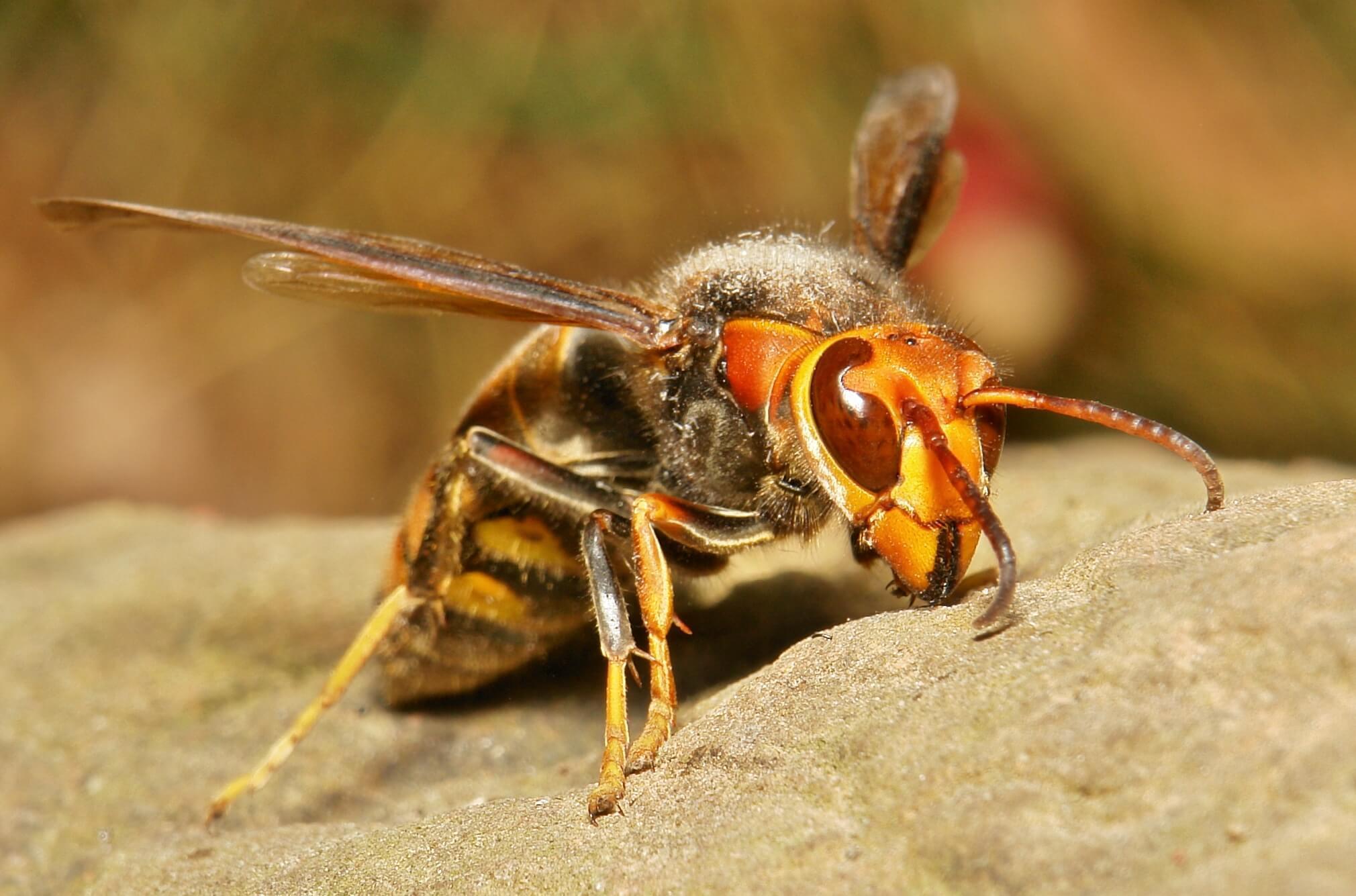The rectangular, horizontally oriented image features a close-up of a honeybee-like insect, prominently situated in the middle. The bee, likely a bumblebee, is perched on a grayish-brown rock material that fills the bottom third of the image. Its head, large and triangular, occupies a central position in the frame and is characterized by huge, oval-shaped eyes, segmented amber-brown antennae, and an orange-ish gold hue with amber and black highlights. Its fuzzy thorax extends outward with two larger, mostly brown wings featuring a black stripe at the front edge, as well as smaller, clearer wings beneath them. The striped abdomen, displaying alternating patterns of yellow and black, stretches behind the thorax. The legs, black and amber/yellow, are clearly visible on one side, adhering to the rock. In the blurred background of the upper third of the image, there's muted brownish coloring interspersed with slight green tones and a red object near the upper right corner, adding depth to the scene.